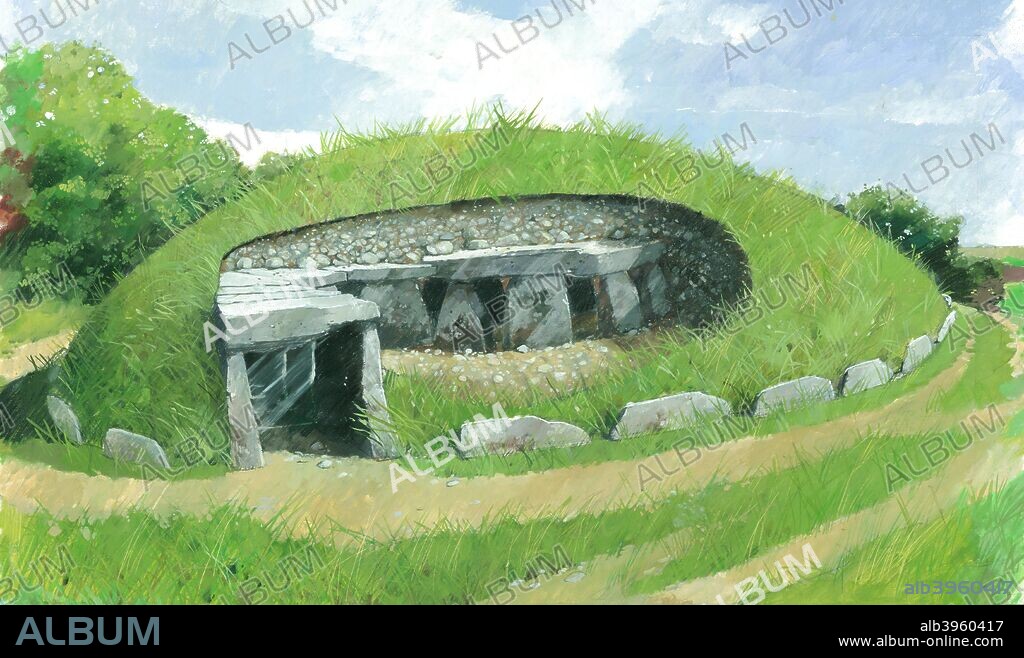The image depicts a detailed colored pencil drawing of a grassy green hill or mound that is adorned with rough-cut stone pillars. At the forefront of the hill, there is a prominent stone-sided doorway with two pillars holding up a slab of stone, suggesting the entrance to a buried tomb or hut. This stone structure appears unfinished and rustic, with additional slabs of stone surrounding the hill, possibly marking the burial site's perimeter. The mound is encircled by a dirt path and flanked by long green grass, adding to the naturalistic feel of the scene. In the background, tall green trees rise up against a bright blue sky dotted with fluffy white clouds. Overlaying the entire image is a translucent watermark bearing the word "album" in white, black, and gray letters. Beneath the image, a black label reiterates the word "album," and to the lower right corner, the text "ALB 3960417" and a website address, www.album-online.com, are visible.